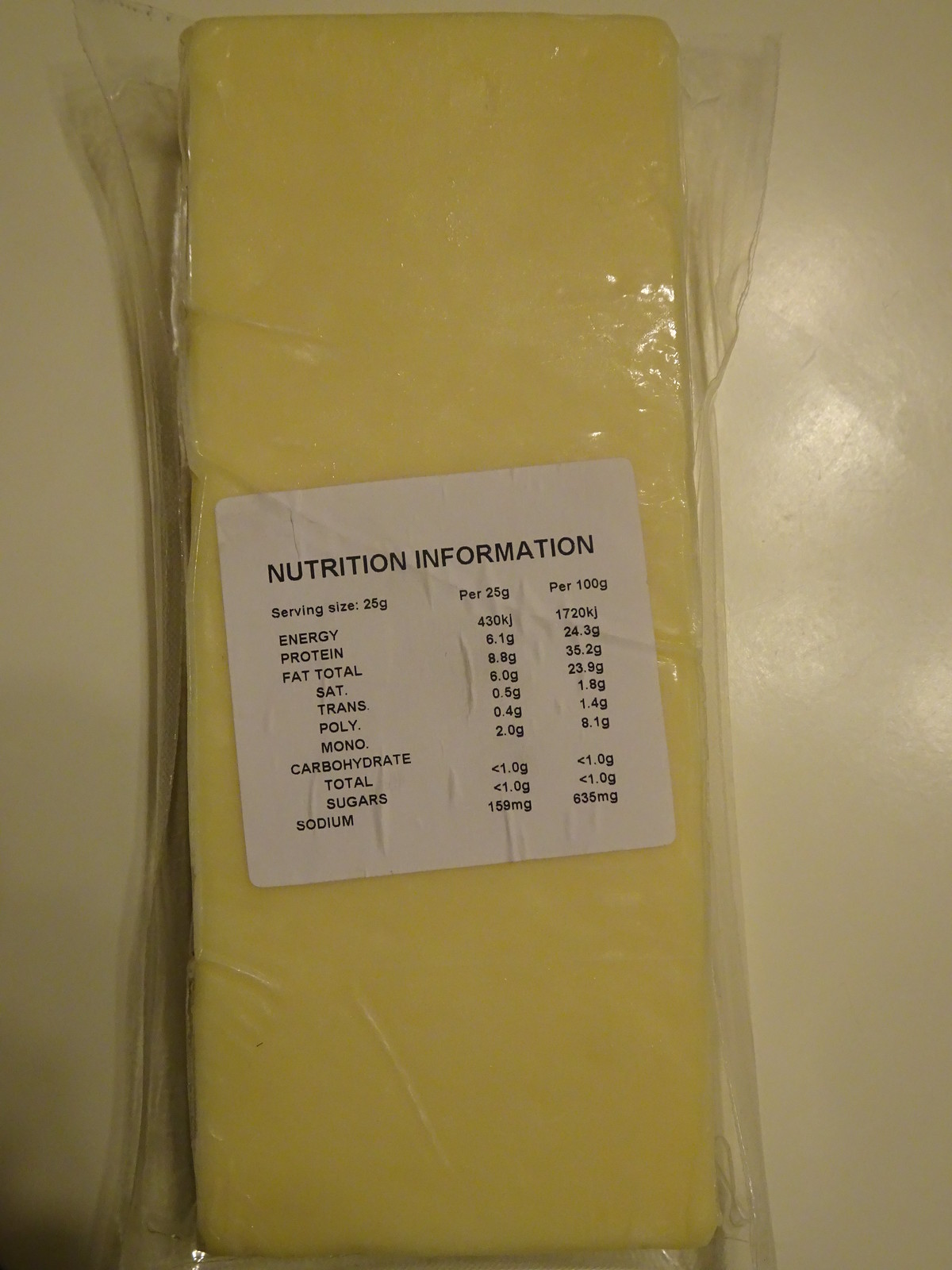This photo showcases a slightly out-of-focus nutrition label affixed to a clear plastic wrapping. The label is presented in a standard white and black color scheme and provides nutritional information, though the details are not fully decipherable due to the image's blurriness. This clear plastic wrapping appears to encase a yellow, rectangular, vertically-oriented object, which might be a block of cheese or similar product. The entire item rests on a white table, providing a neutral background that emphasizes the object and its packaging.